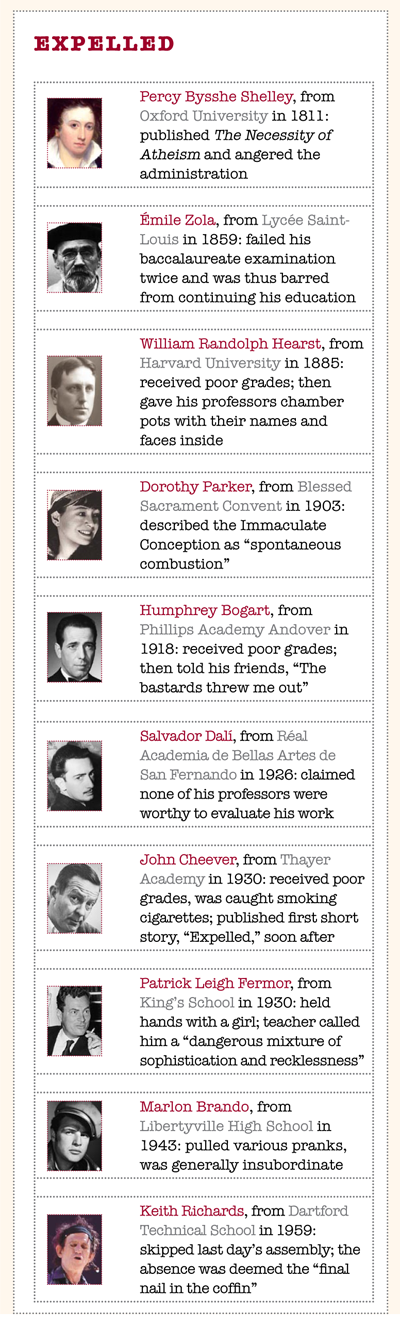The image features a tall table with a series of blocks, each containing a photo and details about individuals who were expelled from various institutions. At the top, in bold red text, it reads "EXPELLED." Each block on the left side shows a thumbnail photo of a person, and on the right side, their name and the reason for their expulsion are detailed.

The first block presents a painting of Percy Bysshe Shelley, who was expelled from Oxford University in 1811 for publishing "The Necessity of Atheism," which angered the administration. The second block has a black-and-white photo of Emile Zola, expelled from Lycée Saint-Louis in 1859 for failing his baccalaureate examination twice, consequently barring him from continuing his education. 

In the third block, a sepia-toned photo of William Randolph Hearst illustrates his expulsion from Harvard University in 1885 due to poor grades, after which he gave his professors chamber pots with their names and faces drawn inside. The fourth block showcases Dorothy Porter, who in 1903 was expelled for describing the Immaculate Conception as a "spontaneous conclusion."

The description continues with Humphrey Bogart, who, in 1918, received poor grades and famously told his friends, "the bastards threw me out," and Balibar Dell, who in 1906 was expelled for claiming none of his professors were worthy to evaluate his work. The list contains several more individuals, each with their own photo, name, and expulsion story, making it a comprehensive catalogue of notable expulsions.